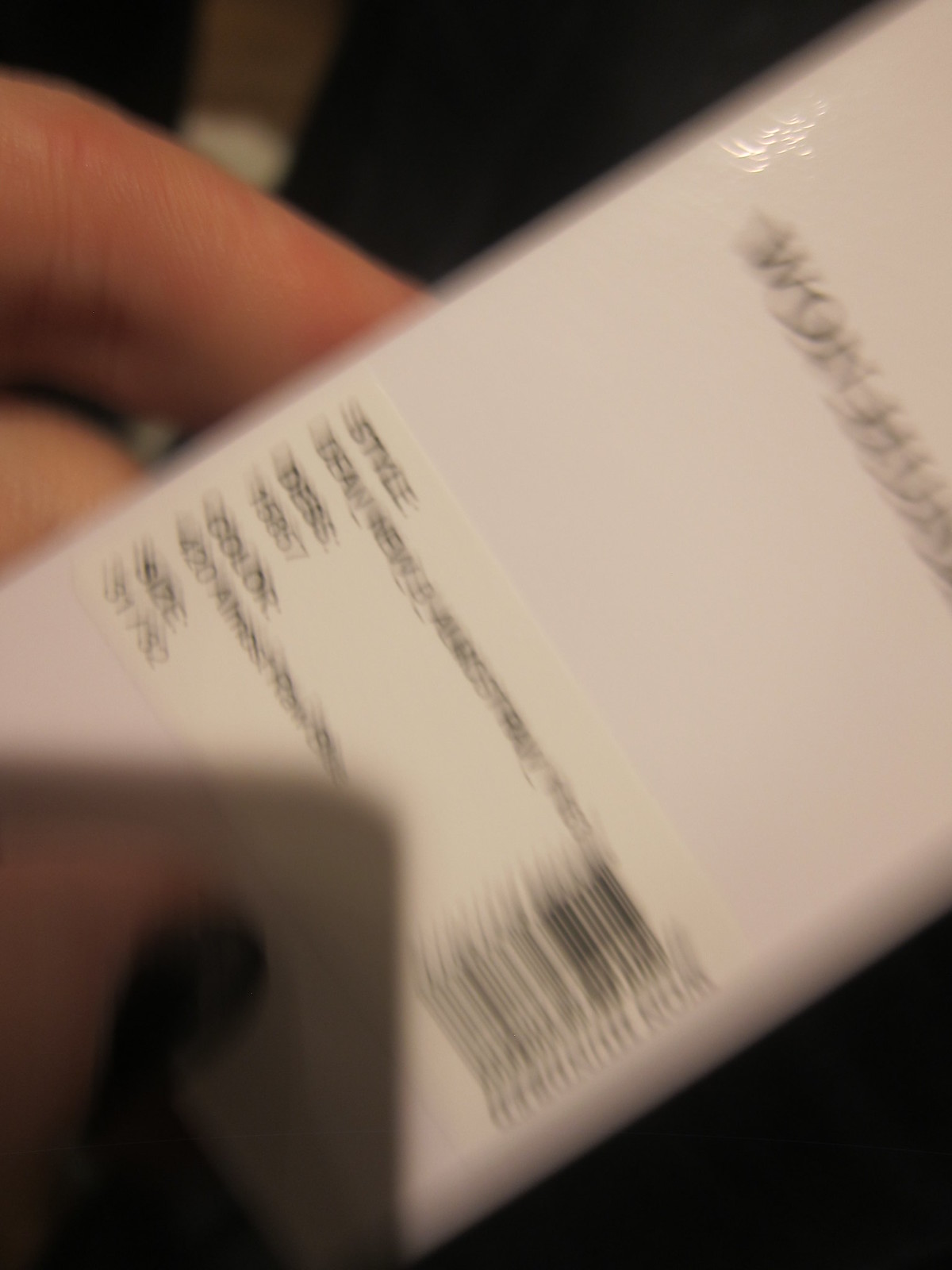This image features a close-up view of a white clothing tag, resembling a price tag. The tag is held by a person's hand, with their index and middle fingers grasping the left side, and their thumb visible at the bottom. The bottom of the tag points towards the lower left corner of the photo, while the top is angled to the right. The tag displays black text at the top and includes a vertical barcode sticker towards the right side, near the bottom. The person's nails, painted in brown polish, are clearly visible. However, the entire photo is out of focus, making the text and details on the tag unreadable.